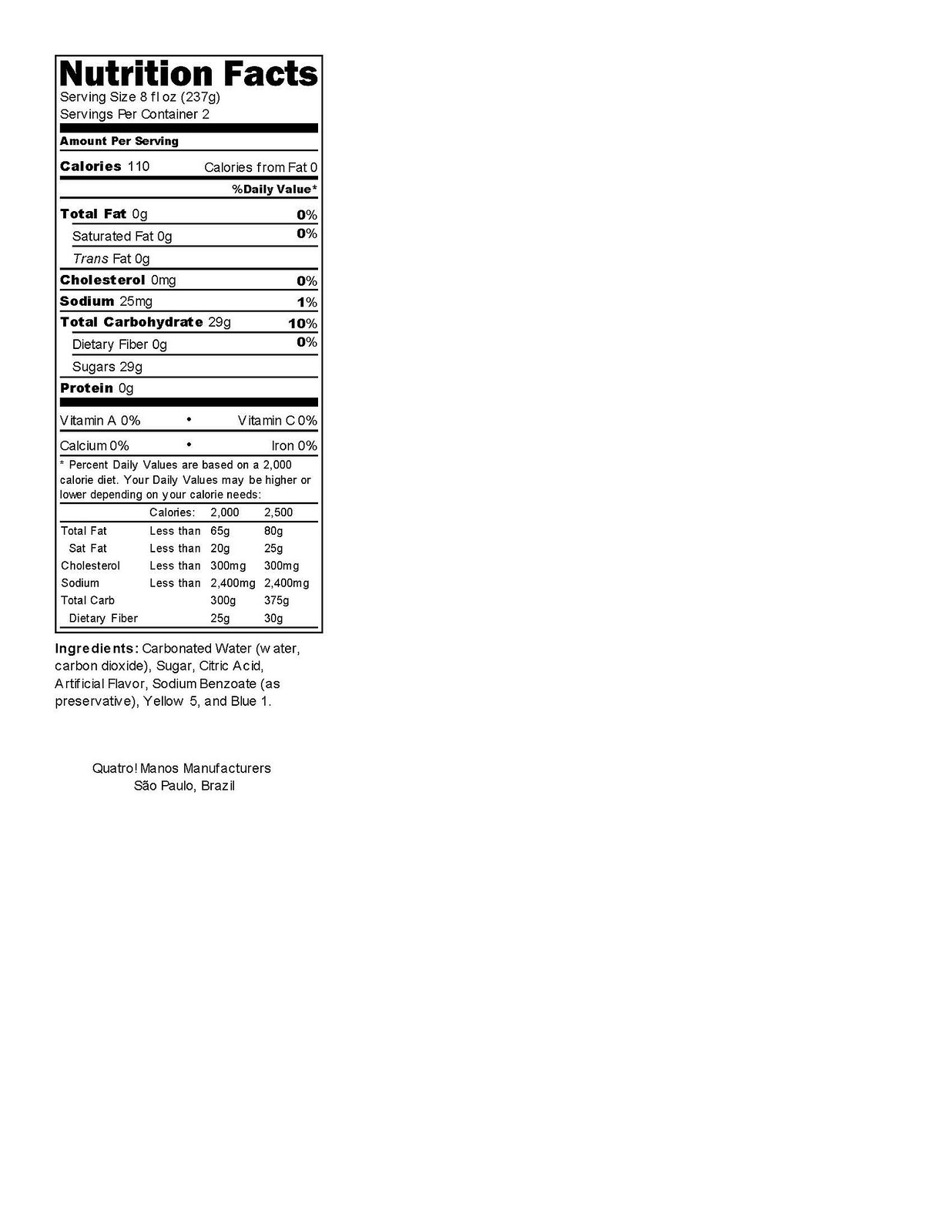The image depicts a large, mostly white background with a black-bordered rectangle containing Nutrition Facts in the top left corner. According to the label, the serving size is 8 fluid ounces (237 grams), with 2 servings per container. Each serving provides 110 calories, with 0 calories from fat. The table lists 0% Daily Value for total fat, saturated fat, cholesterol, dietary fiber, protein, vitamin A, vitamin C, calcium, and iron. It shows 1% Daily Value of sodium (25 mg), and 10% Daily Value of carbohydrates, all from 29 grams of sugar. Beneath the Nutrition Facts, ingredients include carbonated water (water, carbon dioxide), sugar, citric acid, artificial flavor, and sodium benzoate as a preservative, with yellow 5 and blue 1 as color additives. The label mentions Quattro Manos as the manufacturer, based in Sao Paulo, Brazil. There’s also a note stating that the Percent Daily Values are based on a 2,000 calorie diet, with an additional guideline table for calorie needs based on diets of 2,000 and 2,500 calories respectively.